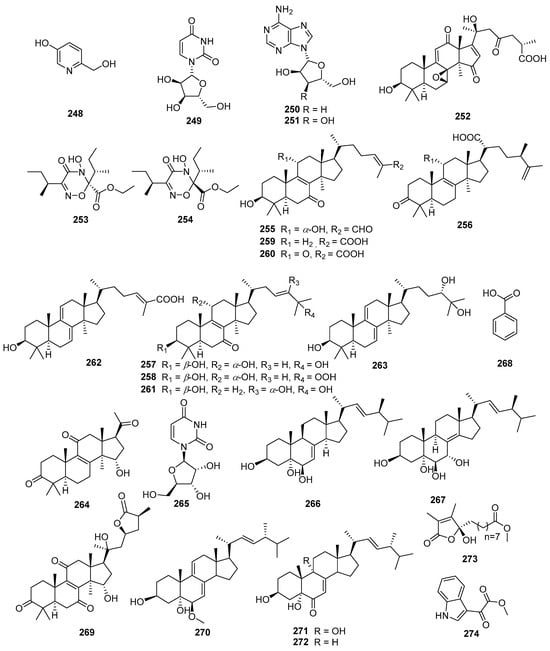This image depicts a page from a chemistry workbook featuring a collection of bond-line formulas for various molecules. The layout includes 5 rows and approximately 4 columns, totaling 20 molecular structures. Each structure is illustrated with black lines representing chemical bonds, and letters denoting elements, predominantly oxygen, nitrogen, and hydrogen. Some of the molecules form hexagonal shapes, indicative of common molecular structures, and these hexagons are often connected by various bonds. The structures span from the upper left-hand corner numbered 248, to the lower right-hand corner numbered 274. Interspersed among the molecular diagrams are chemical equations, with some examples like "R to the 1 equals A minus OH" and "R2 equals CHO." The entire image sits on a plain white background, suggesting it’s a detailed, illustrative page from a chemistry textbook or workbook aimed at illustrating different types of molecular chains and their respective compositions.